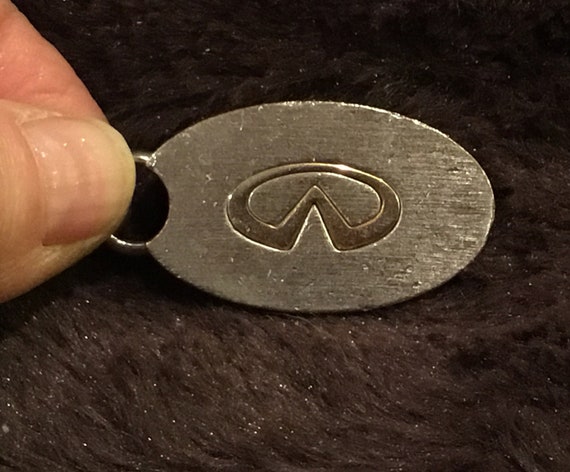The photograph captures a close-up view of a person's thumb and forefinger holding a small, worn metal emblem, most likely a keychain. The emblem is an oval shape made of brushed silver metal and features an infinity car logo, resembling an oval with a central point or an 'A'-like shape. The emblem appears well-used, displaying several nicks and signs of wear from being carried for a long time. The background is blurred and looks like a dirty, sand-specked dark carpet, either black or dark brown. Despite the extreme zoom, the image is remarkably clear, showcasing the meticulous effort put into capturing the detail. The fingers holding the emblem suggest the person is likely white based on their skin tone.